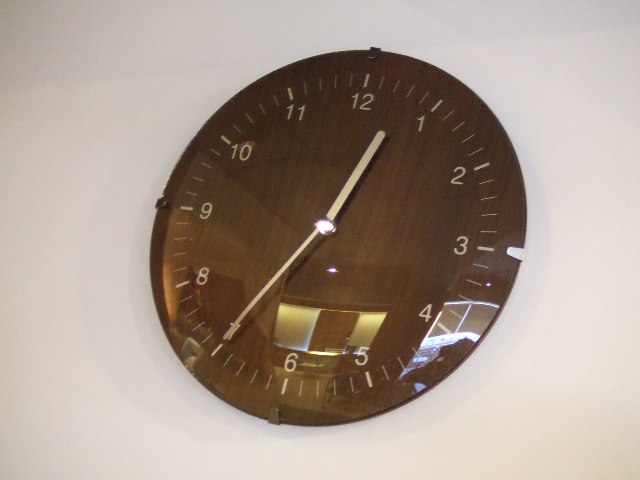A round clock is mounted on a pristine white wall. The clock features a charming brown wood grain face encased in glass, giving it a classic yet polished appearance. Securing the clock to the wall are several metal brackets evenly distributed around its circumference. The numerals on the clock are a soft cream color, matching the cream-colored hands that tell the time. At the center of the clock, a silver bracket holds the hands in place. The glass face of the clock reflects the room's interior; faint images of people are visible along with the glow from a lit projector screen. Additionally, an illuminated object on the left side of the room is also discernibly reflected on the clock’s glass.